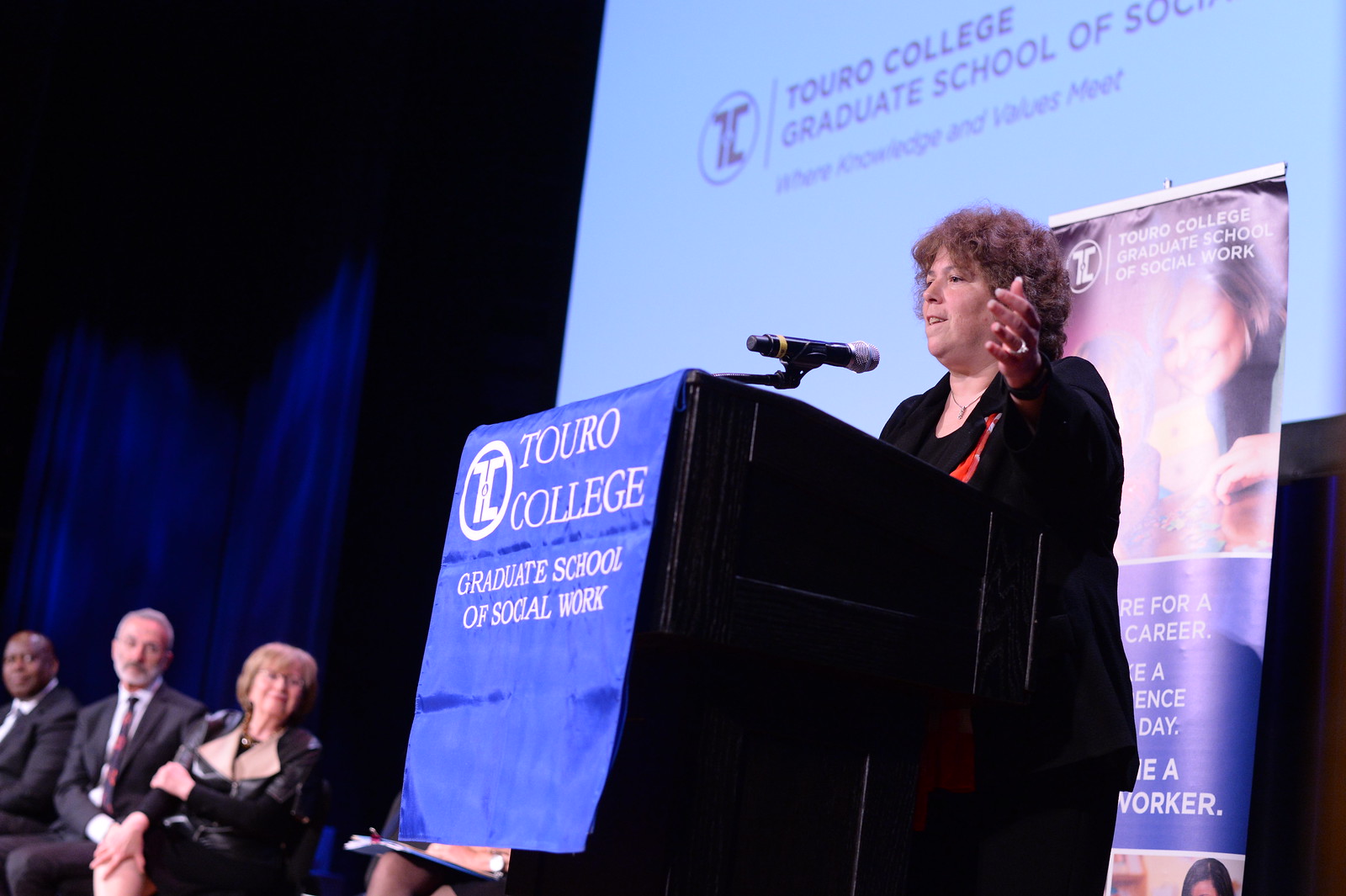The image captures a dynamic scene at the Touro College Graduate School of Social Work. Central to the image is a woman speaking passionately at a black wooden podium draped with a blue cloth that reads "Touro College" in white lettering. Behind her, a large projector screen displays the words "Touro College Graduate School of Social Work" alongside the school's circular T and C logo. The woman, who appears middle-aged with curly brown hair, is dressed in a black blazer and is gesturing with her left hand, emphasizing her speech.

Surrounding her on stage are three other individuals, likely associated with the college: a black man in a suit, a white man also in a suit, and a woman in professional attire. The backdrop of the stage is adorned with a dark blue curtain, creating a formal atmosphere appropriate for what seems to be a graduation commencement. Further adding to the scene's academic ambiance, the banner and screen both highlight the institution's motto, "Where Knowledge and Values Meet," in an off-blue or purplish font against a white background. The overall composition emphasizes the solemnity and importance of the event.